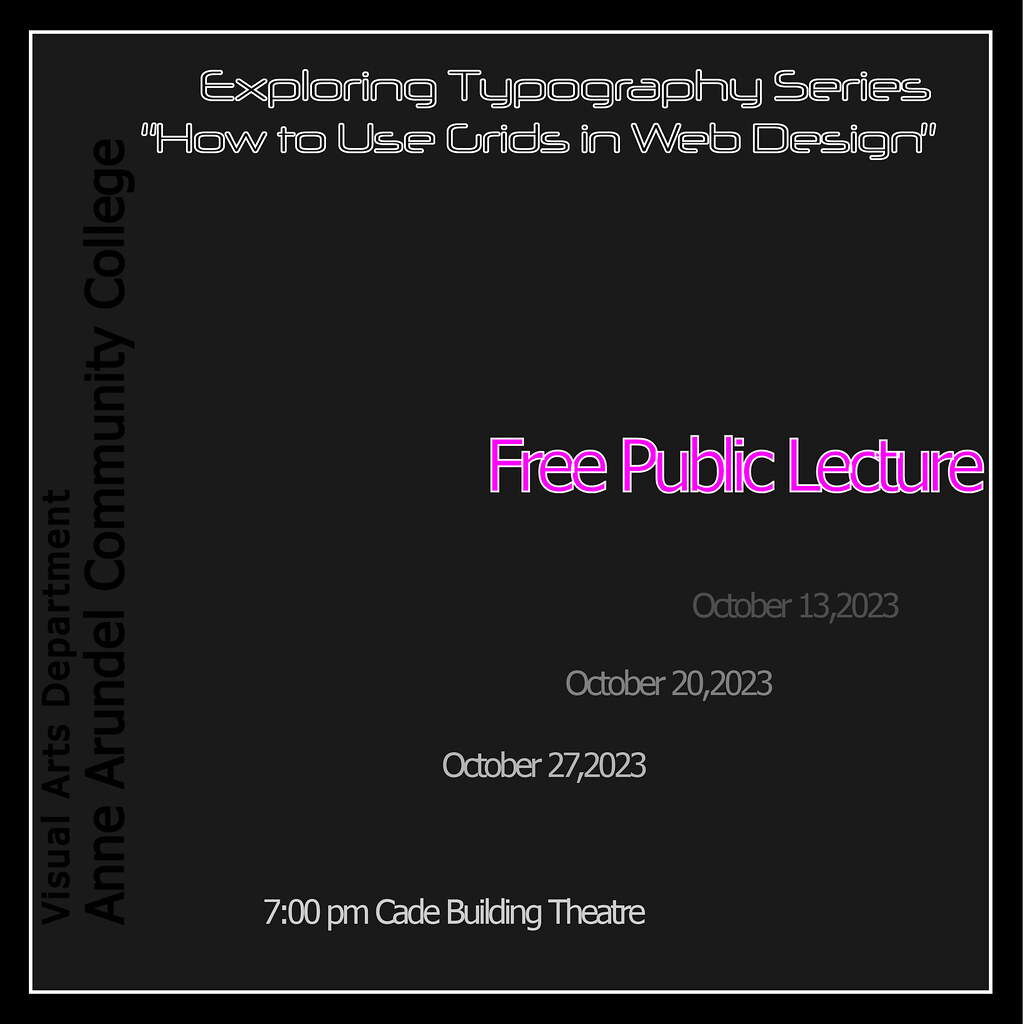The advertisement for an event features a sophisticated design with a gray background and utilizes a color palette of white, gray, red, and green text. It prominently announces the "Exploring Typography Series" at the top in white text, specifically focusing on "How to Use Grids in Web Design." A vibrant red font in the middle highlights the announcement of a "Free Public Lecture." Below this, a gradient of gray to white text lists the event dates: October 13, 2023, October 20, 2023, and October 27, 2023, each taking place at 7 p.m. in the Cade Building Theater. Vertically aligned on the left side in green text, the advertisement credits the Virtual Arts Department of Anne Arundel Community College. The image is framed with a dark brownish-black border and a thin white line, lending a classic, academic feel to the design.